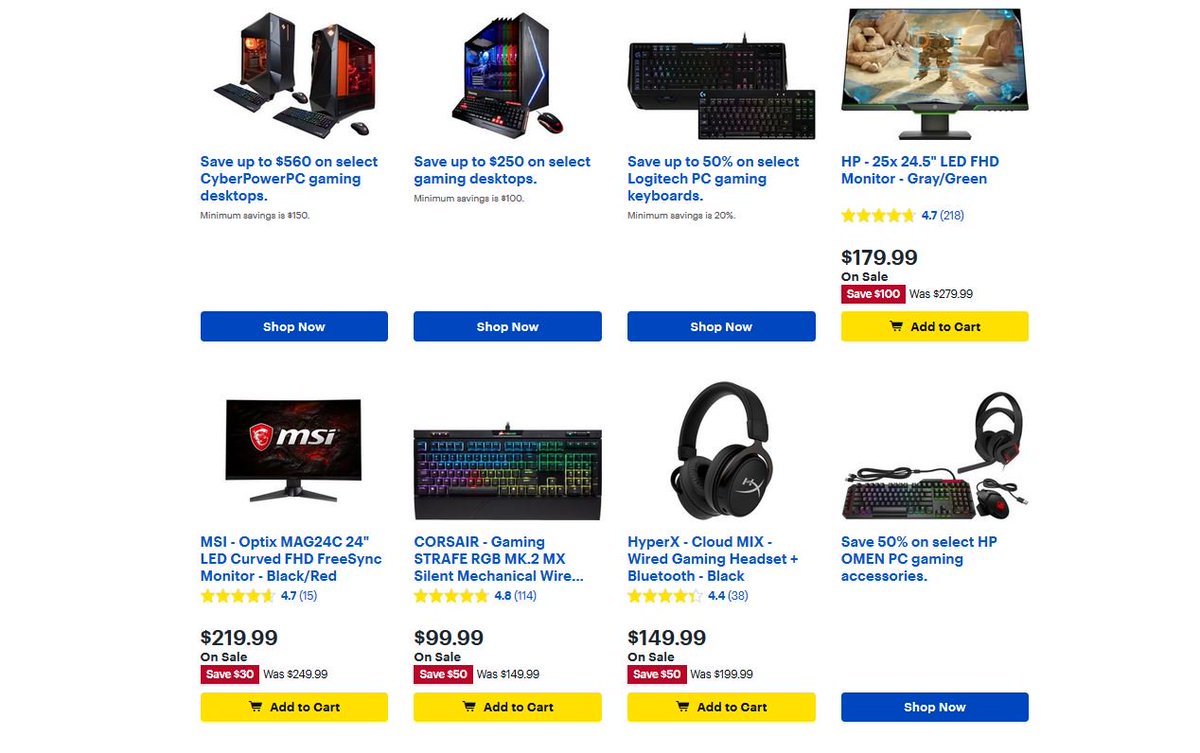This image is a detailed screenshot of a product page from a website that closely resembles Best Buy's, showcasing a total of eight products arranged in two rows of four. Each product listing consists of an image, a title in blue text, and additional information including discounts, ratings, and purchase options.

### First Row Products:

1. **CyberPowerPC Gaming Desktops**
   - **Image:** Two desktop computers, each paired with a keyboard and mouse.
   - **Description:** "Save up to $560 on select CyberPowerPC gaming desktops."
   - **Minimum Savings:** $180.
   - **Button:** A blue rectangle with "Shop Now" in white text.

2. **Gaming Desktop**
   - **Image:** A desktop tower with a keyboard and mouse.
   - **Description:** "Save up to $250 on select gaming desktops."
   - **Minimum Savings:** $100.
   - **Button:** A blue rectangle with "Shop Now" in white text.

3. **Logitech PC Gaming Keyboards**
   - **Image:** Two keyboards; a larger one and a mini version positioned to the bottom right.
   - **Description:** "Save up to 50% on select Logitech PC gaming keyboards."
   - **Minimum Savings:** 20%.
   - **Button:** A blue rectangle with "Shop Now" in white text.

4. **HP 25X 24.5" LED FHD Monitor - Gray and Green**
   - **Image:** LED monitor.
   - **Rating:** 4.7 stars (218 reviews).
   - **Price:** $179.99 with a note of "On Sale."
   - **Discount:** Save $100 in white text on a red rectangle.
   - **Original Price:** Was $279.99.
   - **Button:** A yellow rectangle with "Add to Cart" in black text.

### Second Row Products:

5. **MSI Optix MAG24C 24" LED Curved FHD FreeSync Monitor - Black and Red**
   - **Image:** Curved LED monitor.
   - **Rating:** 4.7 stars.
   - **Price:** $219 with a note of "On Sale."
   - **Discount:** Save $30 in white text on a red rectangle.
   - **Original Price:** Was $249.99.
   - **Button:** A yellow rectangle with "Add to Cart" in black text.

6. **Corsair Gaming Strafe RGB MK.2 MX Silent Mechanical Keyboard**
   - **Image:** Mechanical Keyboard.
   - **Rating:** 4.8 stars (114 reviews).
   - **Price:** $99.99 with a note of "On Sale."
   - **Discount:** Save $50 in white text on a red rectangle.
   - **Original Price:** Was $149.99.
   - **Button:** A yellow rectangle with "Add to Cart" in black text.

7. **Headphones**
   - **Image:** Standard headphones.
   - **Description and pricing details not visible.**

8. **Keyboard, Headset, and Mouse Bundle**
   - **Image:** Keyboard, headset, and mouse set on a white background.
   - **Description and pricing details not visible.**

This well-organized product page provides clear visual and textual details, making it easy to browse and make purchasing decisions for various gaming desktops, monitors, keyboards, and accessories.